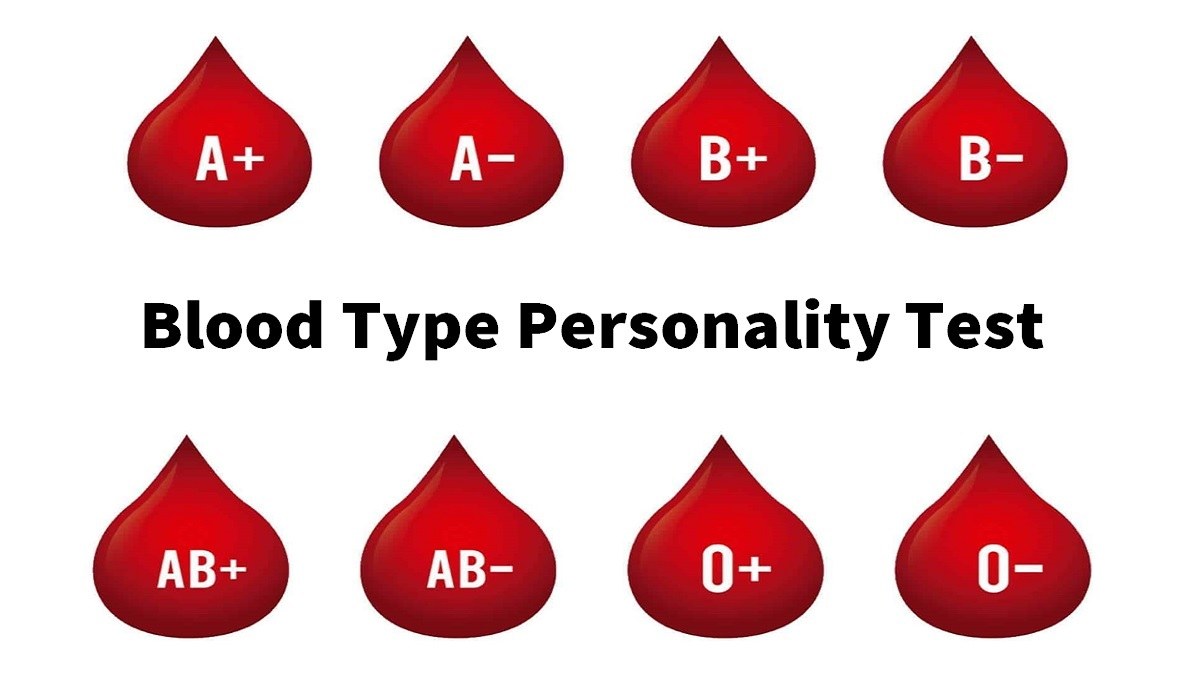The image is a digital illustration resembling a medical diagram with a plain white background. It features eight red blood droplets, each with a black contour and a slight gradient highlight on the left side, arranged in two rows and four columns. The top row consists of droplets labeled A+, A-, B+, and B-, while the bottom row contains droplets labeled AB+, AB-, O+, and O-. Each droplet has white text indicating a different blood type. Central to the image, between the two rows of blood droplets, is a prominent black text that reads "Blood Type Personality Test." This detailed, straightforward design aims to visually communicate the concept of blood type personality traits.